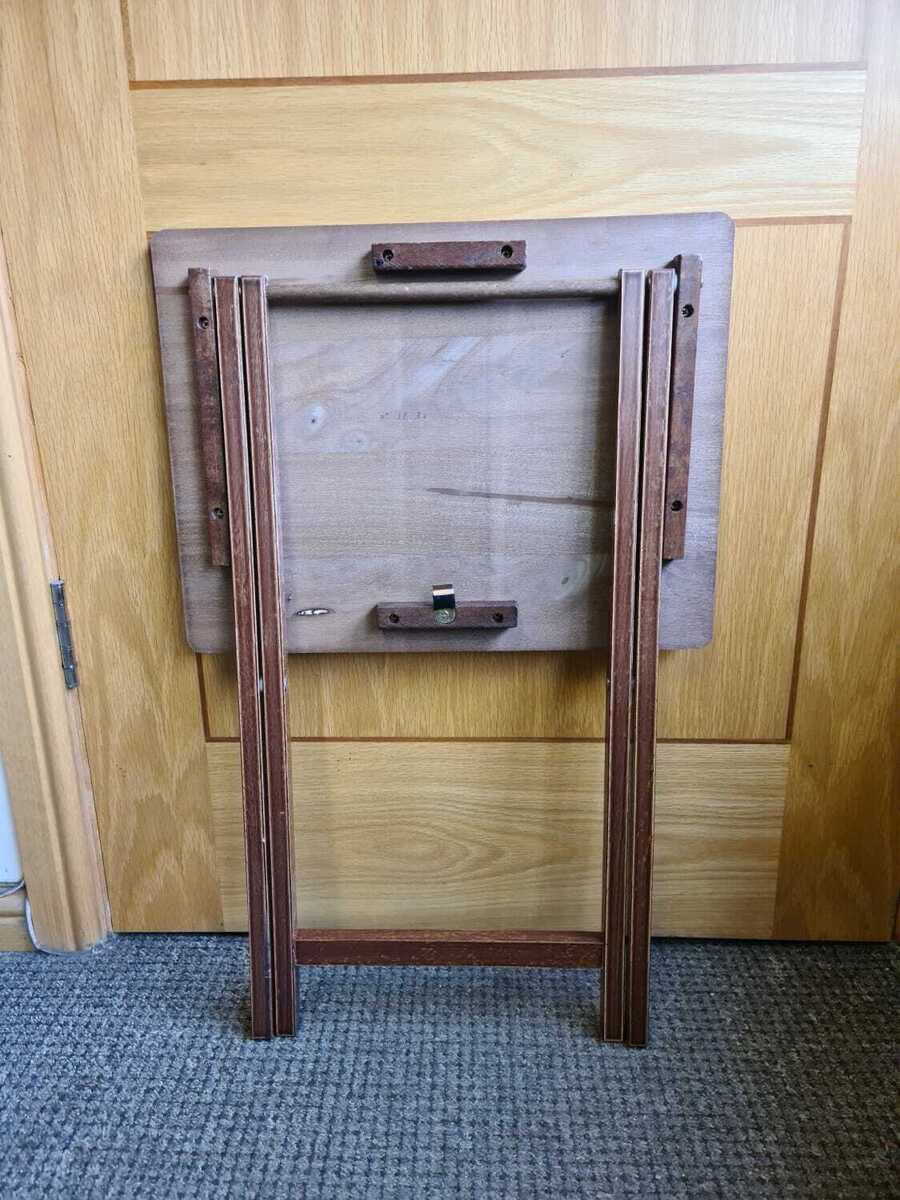In the photograph, a short gray carpet lays on the floor. Resting upon this carpet is a folded wooden table, viewed from its backside. The table's wood showcases a blend of rich chocolatey brown hues alongside paler, more washed-out brown tones. The table leans against a door made of blonde-colored wood, which features darker, chocolatey-colored stripping around its inlays. The grain of the wood on the door is visible, giving it a textured appearance. A pewter-colored hinge is noticeable on the door, adding to the overall rustic aesthetic. The image also reveals a portion of baseboard trim, a sliver of white wall, and a glint of sunlight reflecting off the door, illuminating the scene.